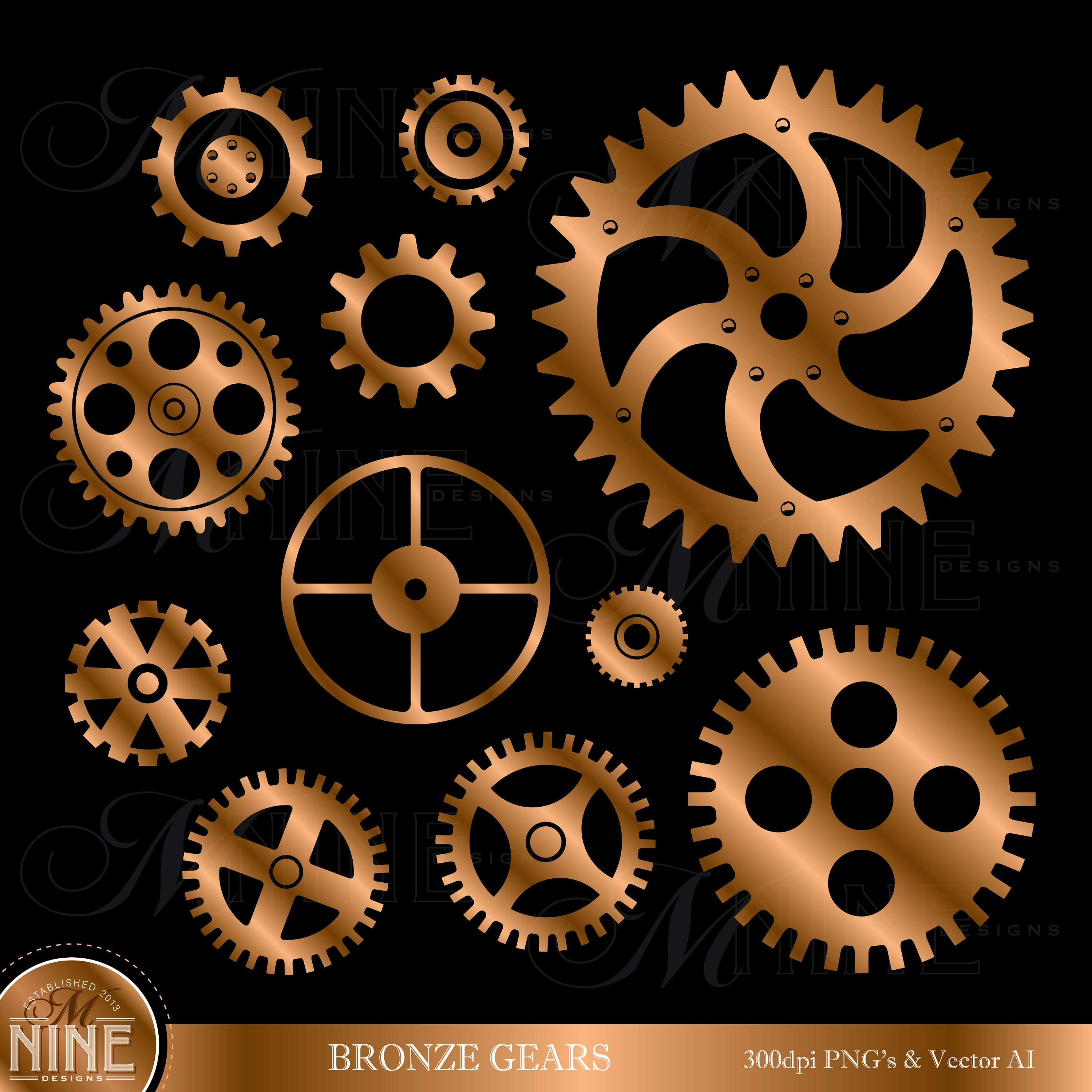This digital illustration depicts a collection of bronze gears set against a stark black background, resembling the intricate mechanisms found inside clocks or watches. The composition meticulously showcases eleven distinct gears, each with varied designs and tooth patterns, illustrating how they would interlock and function together. Some of the gears exhibit intricate details, while others feature simpler, more open constructions. A prominent large gear occupies the top right quadrant of the image, emphasizing the contrast with the smaller gears scattered throughout. Along the bottom, the text in bronze announces "Bronze Gears," accompanied by the logo of Nine Designs, established in 2013. Additional information indicates that the gears are available as 300 DPI PNGs and vector AI files, highlighting the high-quality and versatile nature of the illustrations. This well-crafted poster serves as both an artistic presentation and a functional resource for designers.